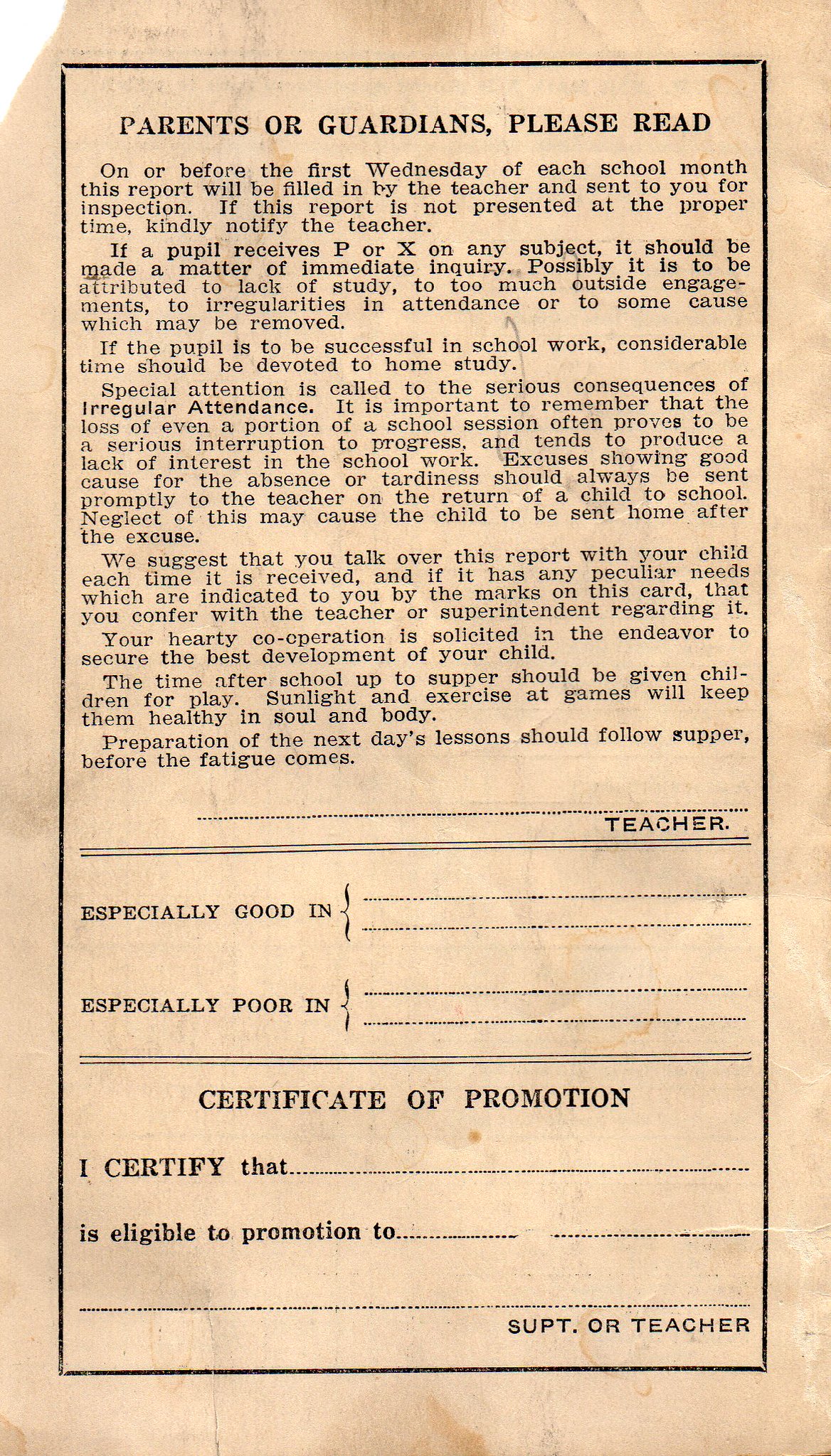This notice, likely from the early 1900s, is printed on aged, yellowing paper and titled "Parents or Guardians, Please Read." It is structured into roughly five sections, some of which feature bolded text to emphasize important points. The notice instructs that on or before the first Wednesday of each school month, the teacher will complete and send this report for parental inspection. Parents are advised to notify the teacher if the report is not received on time.

The notice emphasizes that any pupil receiving a "P" or "X" in any subject should be immediately investigated, potentially indicating inadequate study, excessive outside engagements, or irregular attendance. Irregular attendance is particularly highlighted, noting its serious consequences, such as interruptions to progress and decreased interest in schoolwork. Parents are urged to promptly send excuses for a child's absence or tardiness to prevent the child from being sent home.

The document also suggests parents discuss the report with their child and, if necessary, confer with the teacher or superintendent about any particular needs indicated by the report. Additionally, the notice underscores the importance of balancing play and study: children should have time for play after school and before supper, followed by lesson preparation. The paper includes spaces for teacher and superintendent certifications and signatures, reinforcing the cooperative effort between home and school to ensure the child's best development.